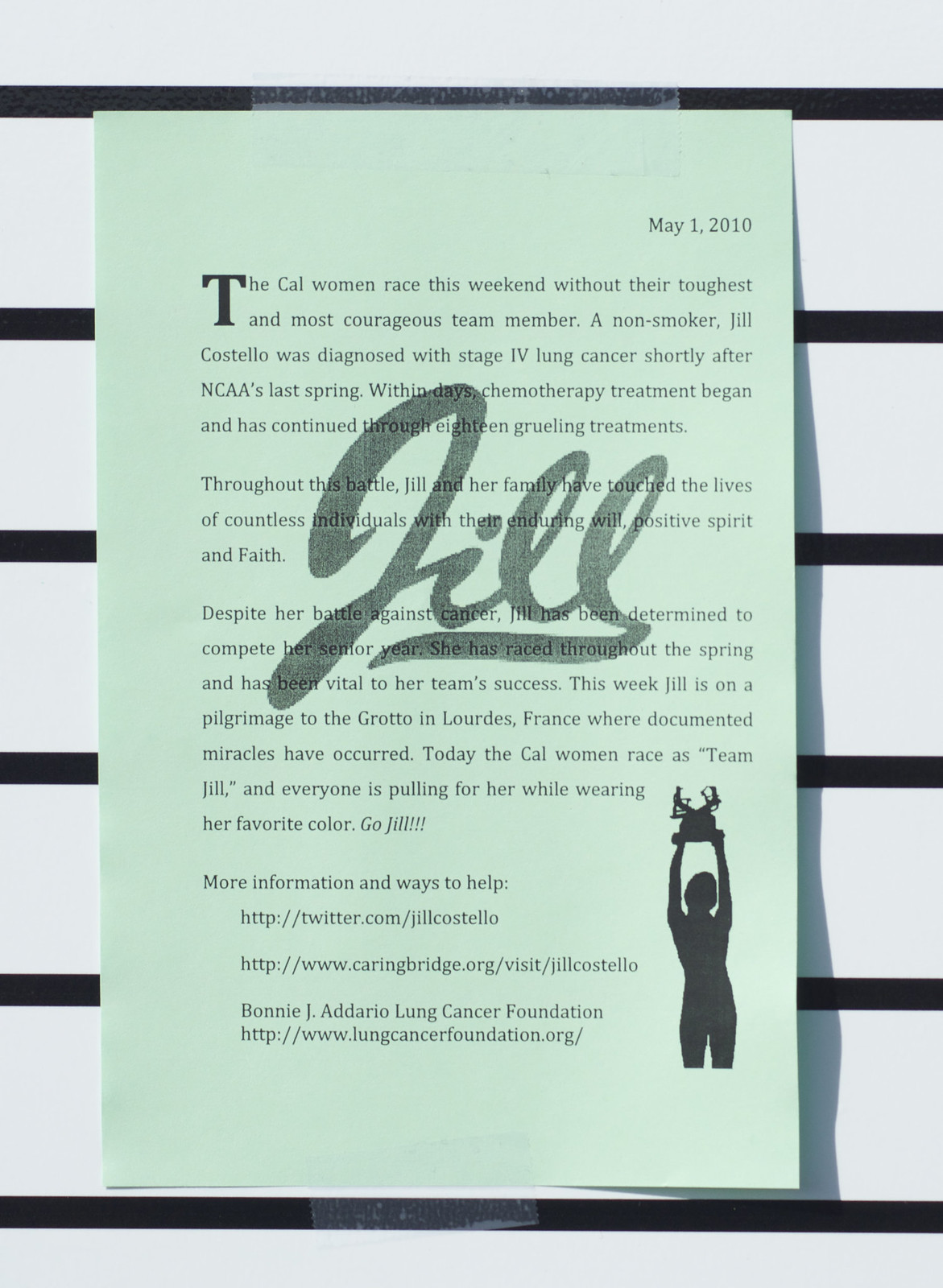A photograph of a teal green piece of paper set against a white background with black horizontal stripes, conveying a heartfelt notice about a woman athlete from the Cal women's team. The paper, dated May 1, 2010, announces that the team will race this weekend without their toughest and most courageous member, Jill Costello, a non-smoker who was diagnosed with stage 4 lung cancer shortly after the NCAA's last spring. Despite undergoing 18 grueling chemotherapy treatments, Jill has continued to inspire others with her enduring will, positive spirit, and faith. She has been determined to complete her senior year and has raced throughout the spring, playing a vital role in her team’s success. This week, Jill is on a pilgrimage to the Grotto in Lourdes, France, where documented miracles have occurred. Today, the Cal women race in her honor as Team Jill, with everyone wearing her favorite color. Written over the text in a transparent outline is the handwritten name "Jill" with a decorative swash, which obscures some of the underlying serif font text. Additional lines at the bottom provide more information and ways to help, alongside two website links that are too small to read. On the right side of the page, there's a silhouette of a woman athlete with outstretched arms holding a trophy above her head. Go Jill!